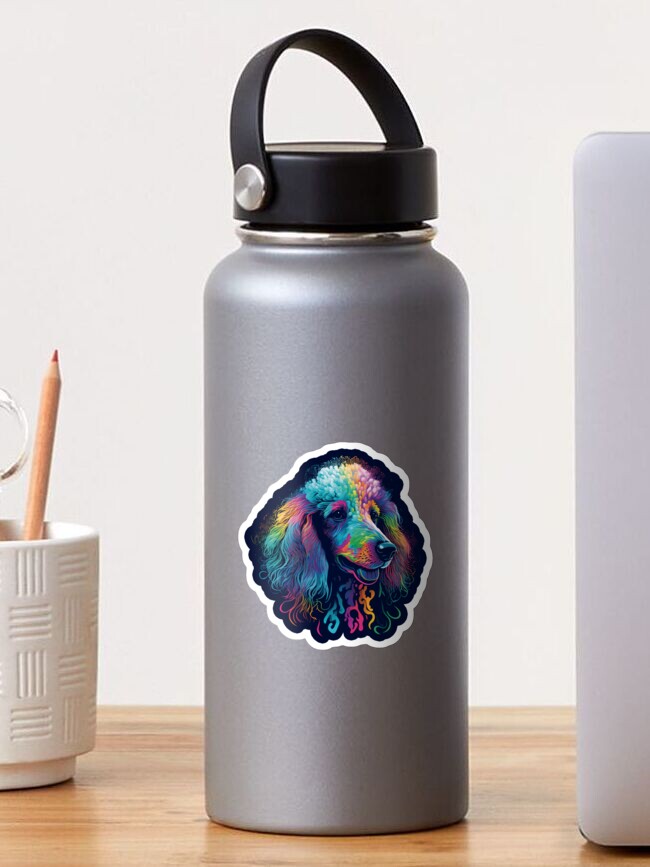This image prominently features a sleek, stainless steel thermos jug, tall and narrow in design, with a capacity suggested to be around 24 ounces. It has a distinctive plastic cap equipped with a handle, firmly attached by a shiny rivet. The thermos is adorned with an eye-catching sticker of a poodle's head that exhibits a psychedelic, multicolored palette reminiscent of a black light painting, with vivid hues of hot pink, orange, blue, and purple against a black background outlined by a white border. The poodle's expressive eyes and fluffy ears stand out, drawing the viewer's attention.

Placed on a wooden countertop, the scene is set against a plain white wall. To the left of the thermos is a white ceramic cup with a tan-colored pencil and partial silver scissors inside, exhibiting distinct vertical and horizontal hash marks. On the right side of the image, a sliver of a silver laptop edge is visible. The photograph overall emphasizes the vibrant and whimsical design on the functional thermos jug within a simple and neat indoor setting.